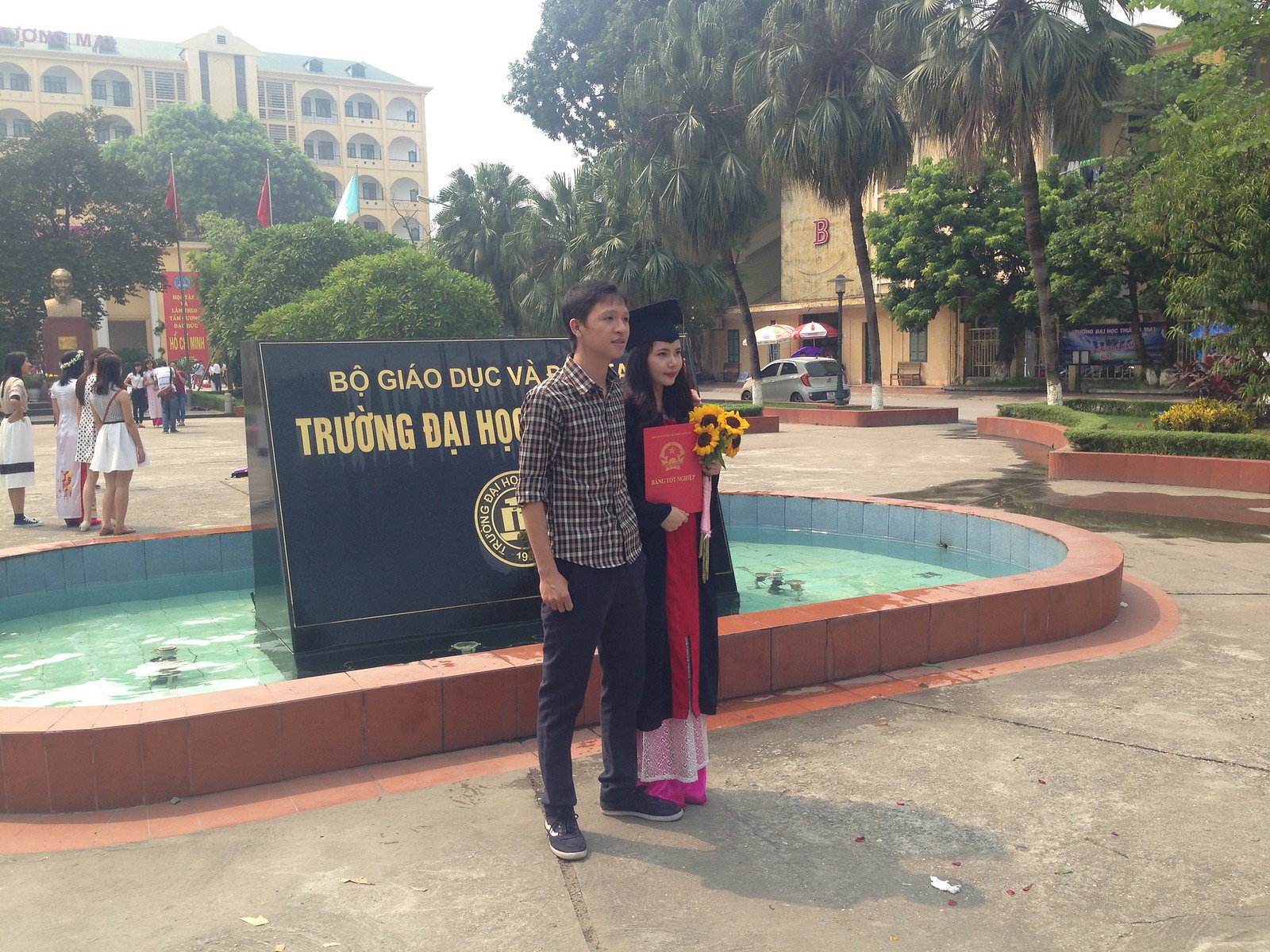The image is a vibrant, landscape-oriented color photograph depicting two young individuals standing on a concrete surface in an outdoor courtyard, in front of an oval brick structure filled with light aqua water. The courtyard features a photographically realistic style focused on representational realism. A large, black monument with gold writing in a foreign language rises from the center of the water behind them.

The main subjects, appearing to be of Asian descent, are a young woman and a young man. The woman, who seems to have just graduated, is dressed in a black graduation gown over a pink and white dress, with a red trim. She wears a traditional graduation cap and clutches a bouquet of bright yellow sunflowers in her left hand and a red diploma with a gold seal in her right. Her shoulder-length dark brown hair frames her radiant expression, suggestive of joy and achievement.

The young man beside her, possibly her brother or partner, has his arm around her in a gesture of support and pride. He is casually dressed in a dark and white plaid shirt with rolled-up sleeves, dark jeans, and dark sneakers. His look is laid-back, contributing to a sense of warmth and connection between the two.

The background includes a bustling plaza with several people scattered around, absorbed in various activities. Beyond the plaza, tall buildings with numerous windows, some with light green roofs, and palm trees contribute to a lively urban landscape. The weather appears to be pleasant, with clear visibility, enhancing the celebratory atmosphere of the photograph. The scene is underscored by details such as a small silver car, red and white umbrellas, and a mix of gray and tan pavements, altogether enriching the context and surroundings of this memorable graduation moment.